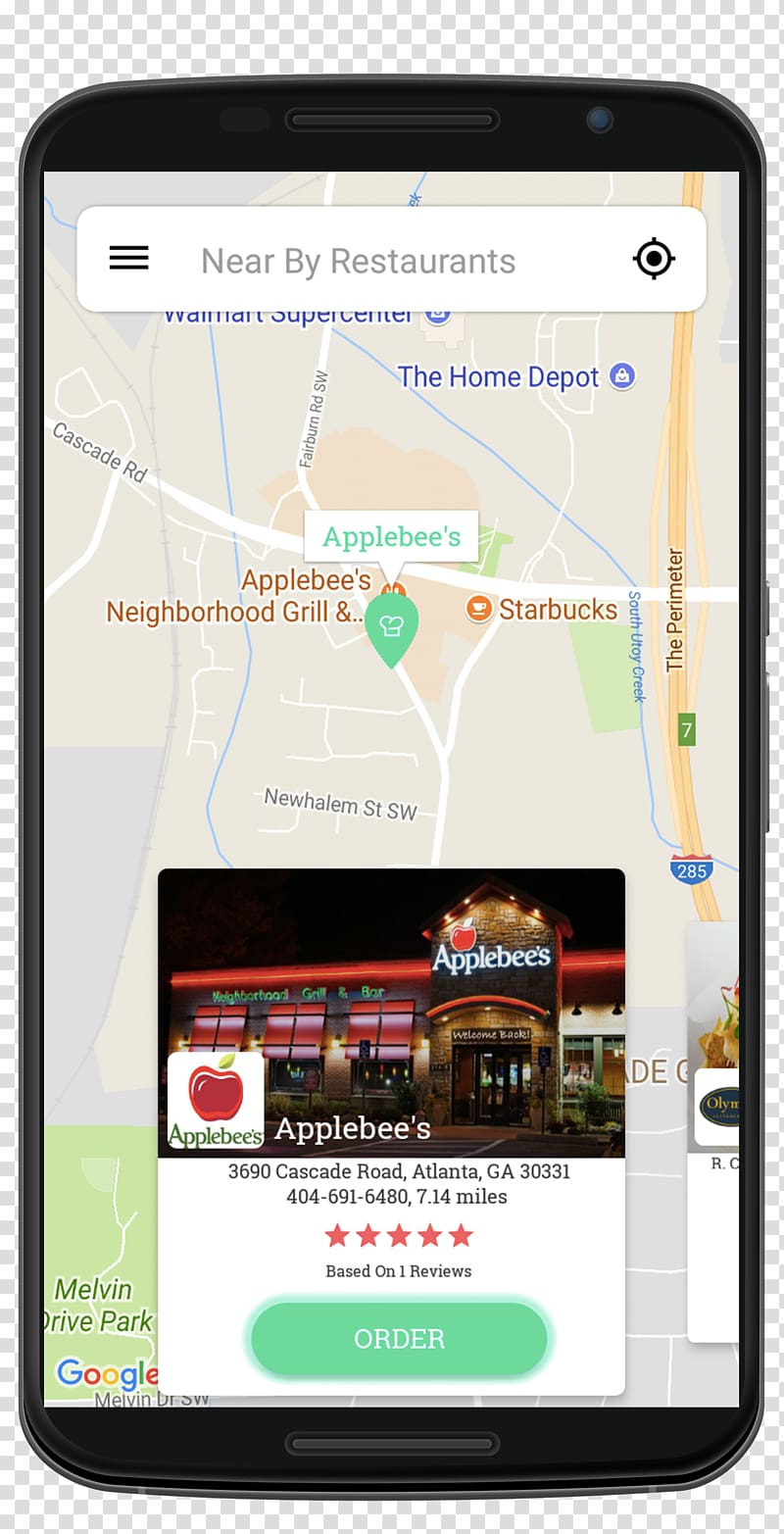The image on this page features a smartphone displaying an app interface. At the top of the screen, there are three black horizontal lines followed by the text "Nearby Restaurants" and a small map icon. Below this header, the screen is dominated by a map, with an Applebee's restaurant highlighted at the center. The map pin for Applebee's includes an image showing the front view of the restaurant, along with the Applebee's logo. Detailed information below the logo provides the address: 3690 Cascade Road, Atlanta, Georgia 30331, along with a contact number: (404) 691-6480. The distance to the restaurant is listed as 7.14 miles. Additionally, the restaurant has received a five-star rating based on one review. A green button labeled "Order" is prominently displayed for convenient access. The background of the phone screen features a black-and-white checkered pattern with alternating gray and white squares.